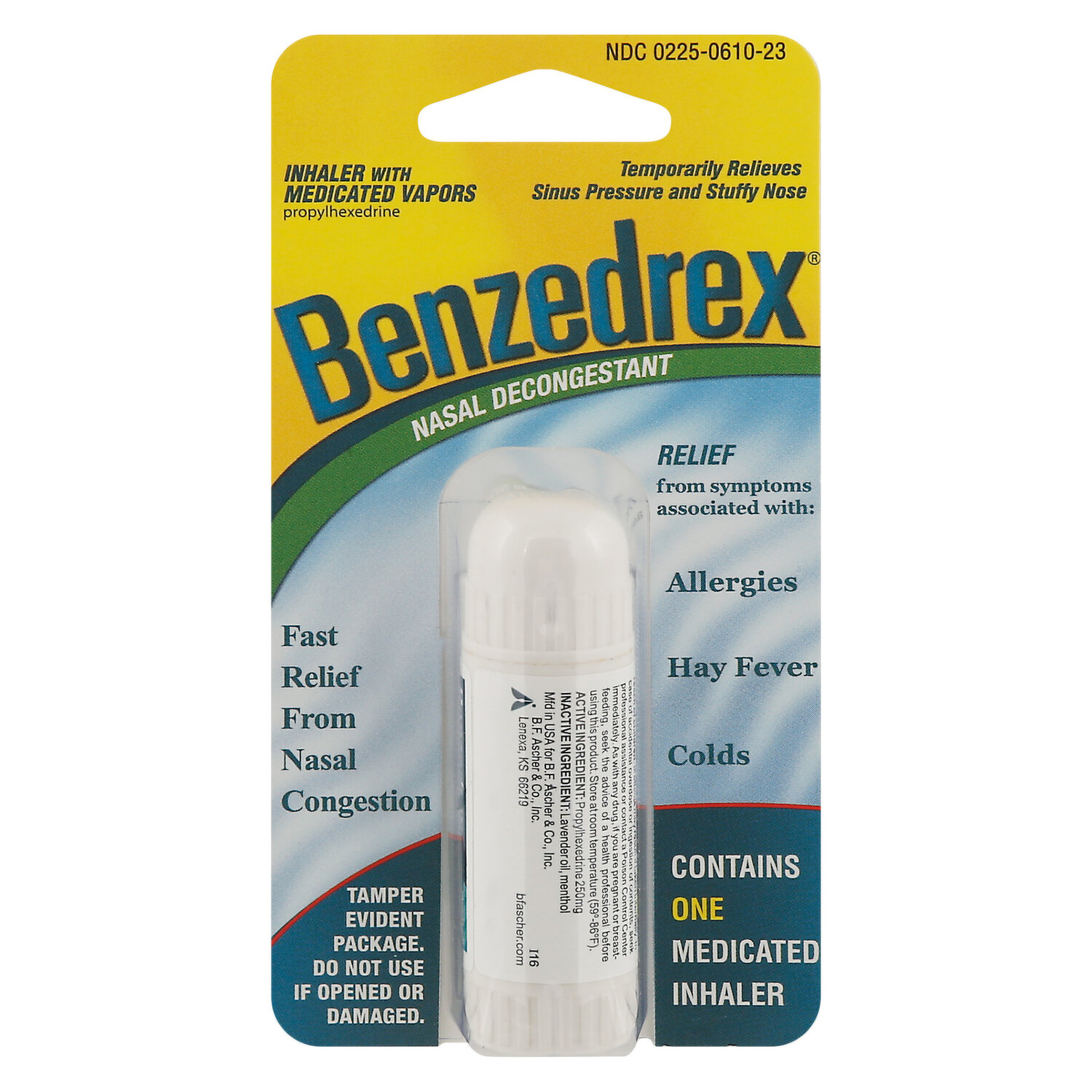This is a color photograph of the product packaging for Benzedrex, a nasal decongestant inhaler with medicated vapors. The rectangular cardboard package features a cylindrical white medicated inhaler in a plastic blister pack at the bottom center to the middle center. The top section of the package is yellow with the brand name "Benzedrex" and "nasal decongestant" prominently displayed. Below this, the middle section is light blue, containing dark blue text: "Fast Relief from Nasal Congestion" on the left, and "Relief from Symptoms Associated with Allergies, Hay Fever, Colds" on the right. The bottom portion is dark blue, stating "Contains 1 Medicated Inhaler." It also emphasizes its tamper-evident design with the warning, "Do not use if opened or damaged." The white inhaler itself is described as offering temporary relief from sinus pressure and stuffy nose, with additional text indicating the active ingredient, propylhexedrine. The overall design of the cardboard package integrates yellow, light blue, and dark blue hues, ensuring clear visibility of the product and its benefits.